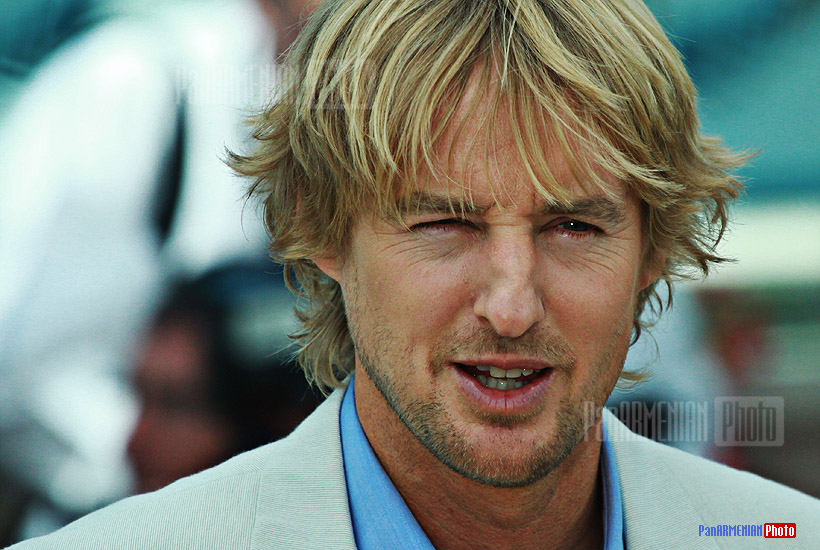This horizontally aligned, wide rectangular image features a close-up of a Caucasian man from the shoulders up, fading into the image's bottom. The man's disheveled, short, shaggy blonde hair, highlighted with darker tones, frames a face with tan white skin and a ruddy neck. His expression is marked by a slight smile, revealing somewhat crooked teeth from both rows. He also sports a bit of stubble, with a blonde mustache and a light blonde beard. His crooked nose tilts to the left. Due to squinting, his left eye is nearly closed, while his right eye is only slightly visible. 

He wears a white suit jacket over a bright blue collared shirt. The background is a complex blend of blurry colors and shapes, including teal, pink, and various blobs of white and black. Behind him are two blurry white objects or one split by a thin black vertical gap, diagonally aligned. To the upper right, a pink triangular shape points off to the top right with some additional vibrant hues scattered around.

Superimposed in faint, narrow capital letters, "Pan-Armenian" appears on the left side, while a small white rectangle with "photo" written on it in gray font is positioned to the right. In the lower right corner, "PHOTO" appears in white font over a small red rectangle. The photograph's style, potentially from the early 2000s, might be linked to the actor's popularity during that time.